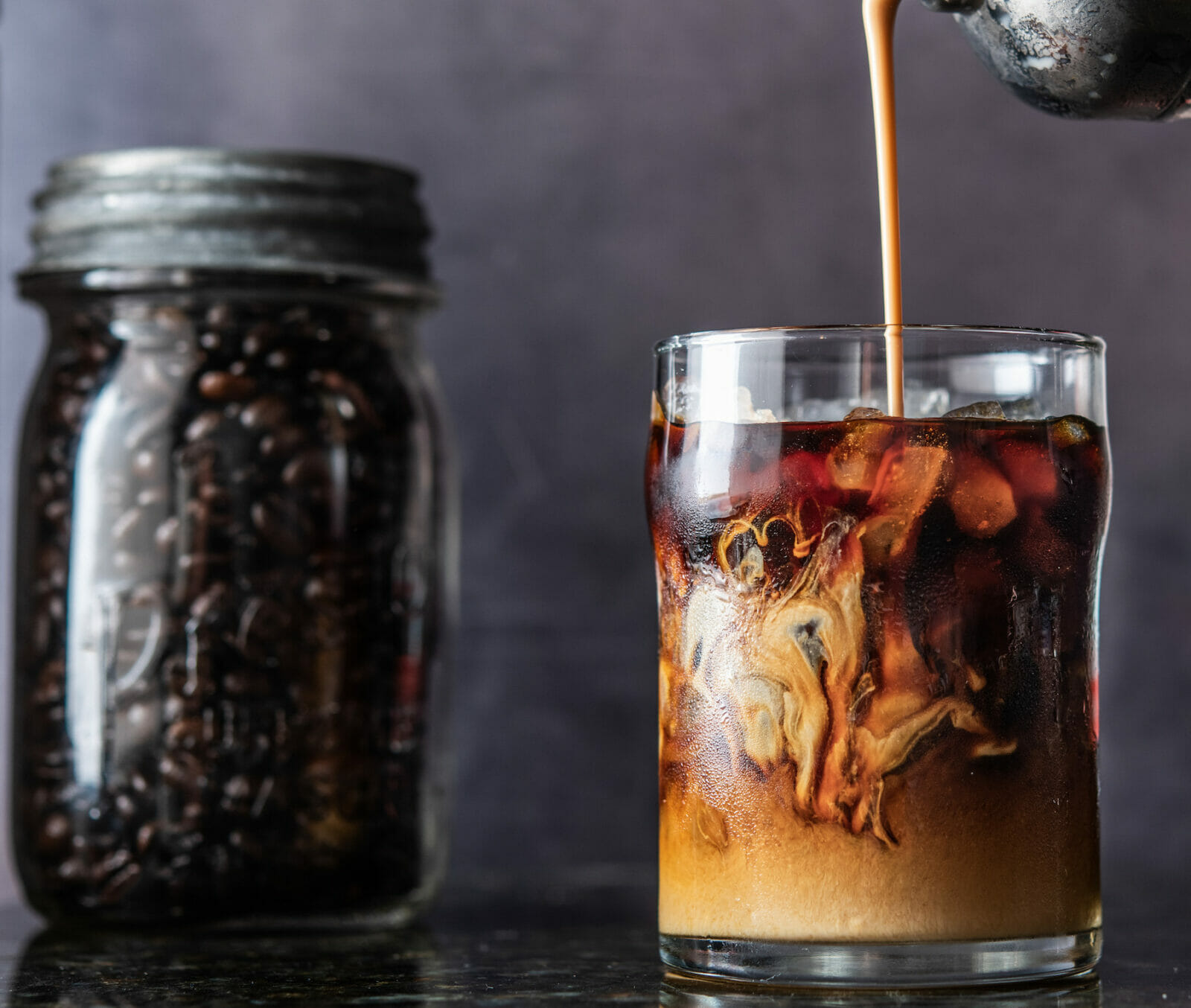In the image, a glass of iced coffee is being poured with a creamy, light brown liquid from a silver container. The clear glass displays a mesmerizing mix of colors, with the iced coffee exhibiting a brownish-red hue at the top and a white and light brown blend at the bottom, separated by swirls where the two shades meet. The ice cubes float at the top, adding to the visual appeal. The drink is set on a sleek, dark almost marble-like countertop. In the background, against a grayish wall, sits a mason jar filled to the brim with coffee beans, slightly out of focus. The jar has a silver metal lid and adds an element of rustic charm to the scene.